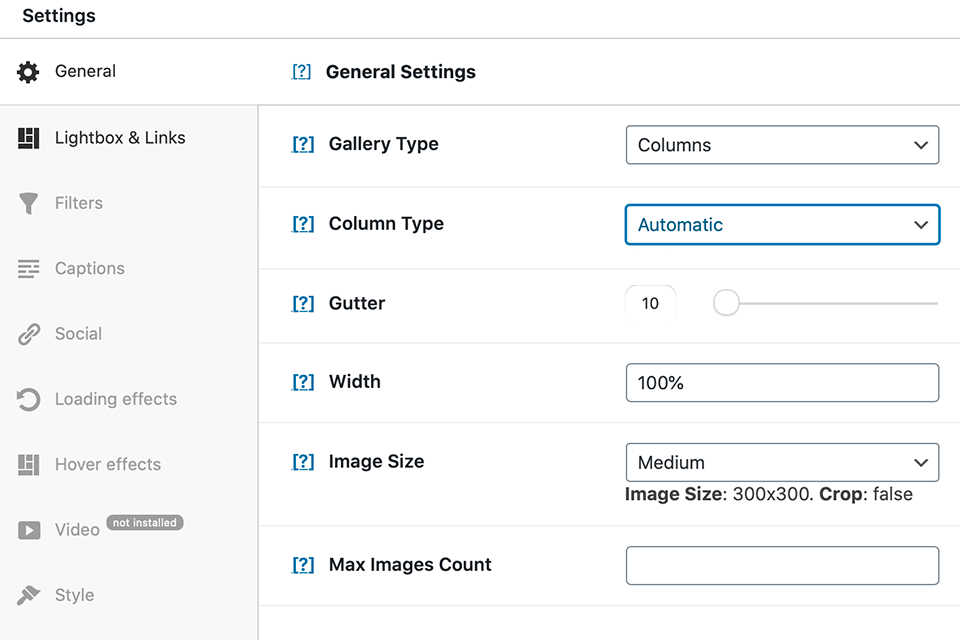The image depicts a detailed interface for configuring settings, likely of a gallery or content management system. 

At the top left, the word "Settings" is displayed prominently in bold text. Directly below this heading, a light-colored horizontal line runs from left to right, serving as a separator for the subsequent sections.

The first section features an icon of a settings wheel adjacent to the word "General" in black font. Proceeding to the middle column, there's a blue-outlined square with no top. Inside this square, a blue question mark is set against a white background. Below this, the phrase "General Settings" appears in bold black font. Another horizontal line, identical to the first, separates this entry from the next.

On the left side, the background is light gray and displays a vertical list of items, each preceded by an icon. These items include: 
- Lightbox
- Ampersand
- Links
- Filters
- Captions
- Social
- Loading Effects
- Hover Effects
- Video
- Style

Notably, "Lightbox" and "Links" are in bold black font, while the rest are in gray font.

To the right of this list, in black bold text, are additional options, each paired with a blue question mark in a box to the left. These options are:
- Gallery Type
- Column Type
- Gutter Width
- Image Size
- Max Images Count

Moving further right to the third column, there are several horizontally arranged fields with white backgrounds:

1. The first field displays the word "Columns" in black font with a pull-down menu to the right.
2. The second field states "Automatic" in blue text with a blue outline around the box and a black pull-down menu.
3. The third field contains a little horizontal oval with the number "10" inside, accompanied by an on-off switch that appears to be in the off position (all the way to the left).
4. The next field reads "100%" and is followed by another option, "Medium," with a pull-down menu to the right.
5. Under this, the following text is shown in black bold font: "Image Size," followed by "300 x 300" in regular black font.
6. Below, "Crop" is in bold black font, adjacent to the word "False," which is in regular black font.
7. The final field in this column is empty.